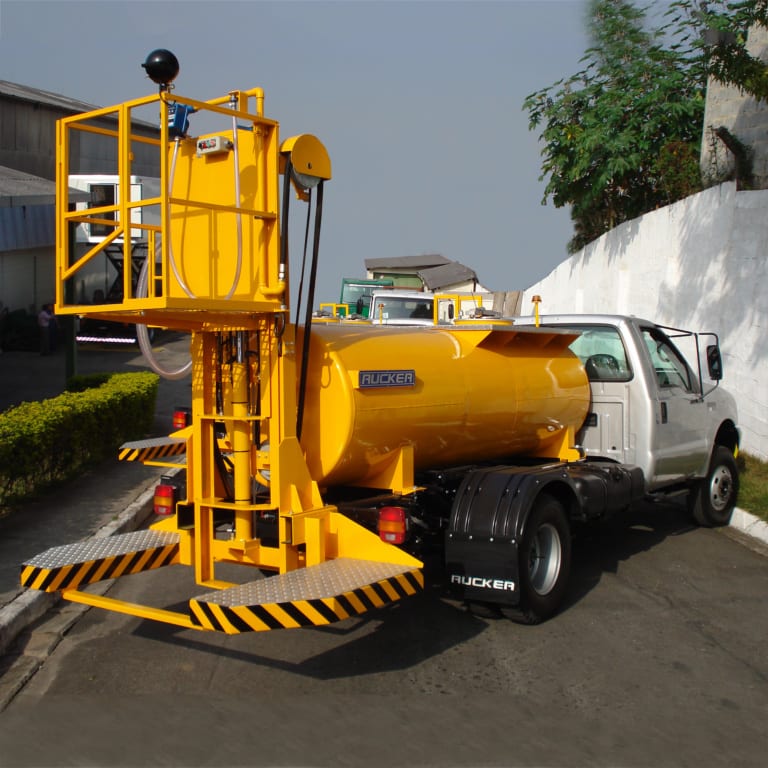The image depicts a white or silver industrial truck with a flatbed trailer, seen parked diagonally along a curb near a tall white wall with overhanging greenery. The truck features a prominently placed cylindrical yellow tank labeled "Rucker," designed to hold liquids such as fuel or chemicals. Attached to the end of the tank is a bright yellow platform elevator, resembling a man lift or cherry picker. This elevator has a grated metal surface and is equipped with a caged platform and a large black circular knob at the top, allowing for vertical movement. Additional safety features include spaced-out large silver feet with yellow and black caution striping. The truck cab, capable of seating two, is angled lower on the left and higher on the right against a backdrop of green shrubbery and buildings. The sky above is a light blue-gray, clear of clouds.